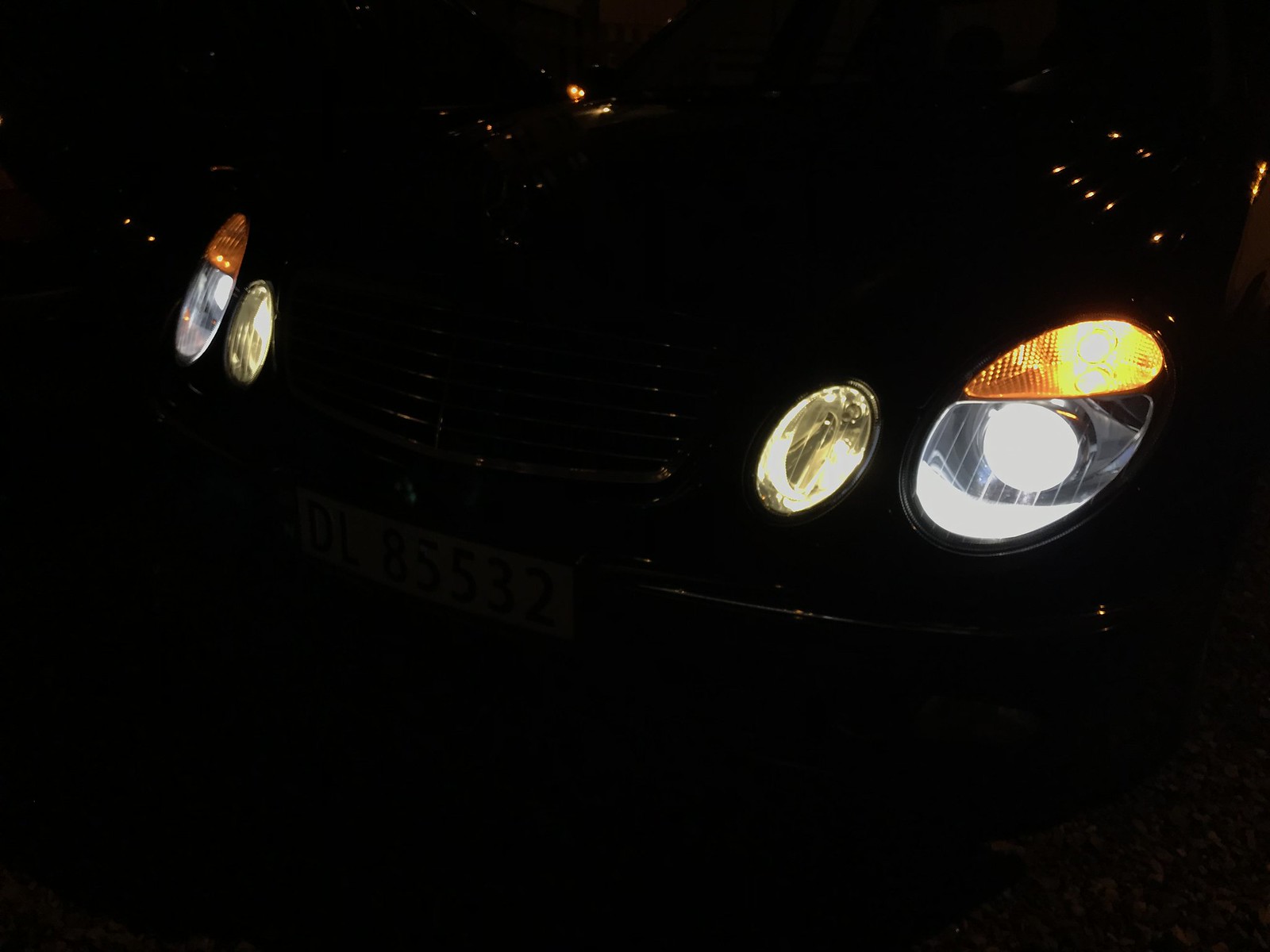In this nighttime photograph, the front of a black car is captured against a completely dark background, with the car itself barely visible except for its gleaming headlights and certain light reflections on its hood. The car features four distinctive headlights. On each side of the car, there is a prominent oval-shaped headlight that emits a clear white light. Above each large oval headlight, there is a smaller, pear-shaped yellow light with ridges, acting as a reflector. The leftmost and rightmost headlights are also characterized by additional oval-shaped yellow lights above them. The vehicle appears to have a unique license plate reading "DJ-85537," indicative of an overseas registration. The focus of the image is clearly on the illumination provided by the headlights, which stand out starkly against the darkness.